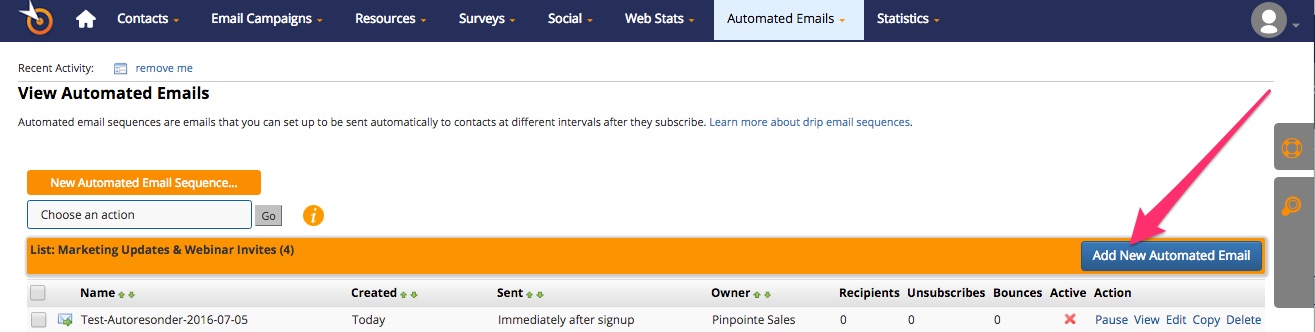The image showcases the layout of a website interface, detailing various components and functionalities. The interface appears to be for managing email campaigns and automated sequences.

In the upper right-hand corner, there is an orange circle with another orange circle in the middle and a white arrow on the side, presumably representing the company's logo.

Below the logo, there are several navigation options that include: Contacts, Email Campaigns, Resources, Survey, Social Web Stats, and Automatic Emails & Statistics. Moving to the right side of the interface, there is a generic icon of a circle containing a white silhouette of a person, which appears alongside the option to "View Automatic Emails."

The section elaborates on automated email sequences, which can be set up to be sent automatically to contacts at varied intervals after they subscribe. There’s a clickable blue text link that says "Learn more about original email sequences."

Beneath this information, there is an orange bar containing the text "New Automated Email Sequence". Users can choose an action within a white bar labelled "Marketing Updates and Webinar Invites." Within this orange bar, there is also a red arrow pointing directly to the text "Add New Automated Emails."

Finally, the interface lists details such as Name, Created, Sent, Owner, and Recipients, indicating that these fields are filled out and presumably represent specific email sequences that have been set up.

This detailed description captures the user interface elements and functionalities of the website shown in the image.